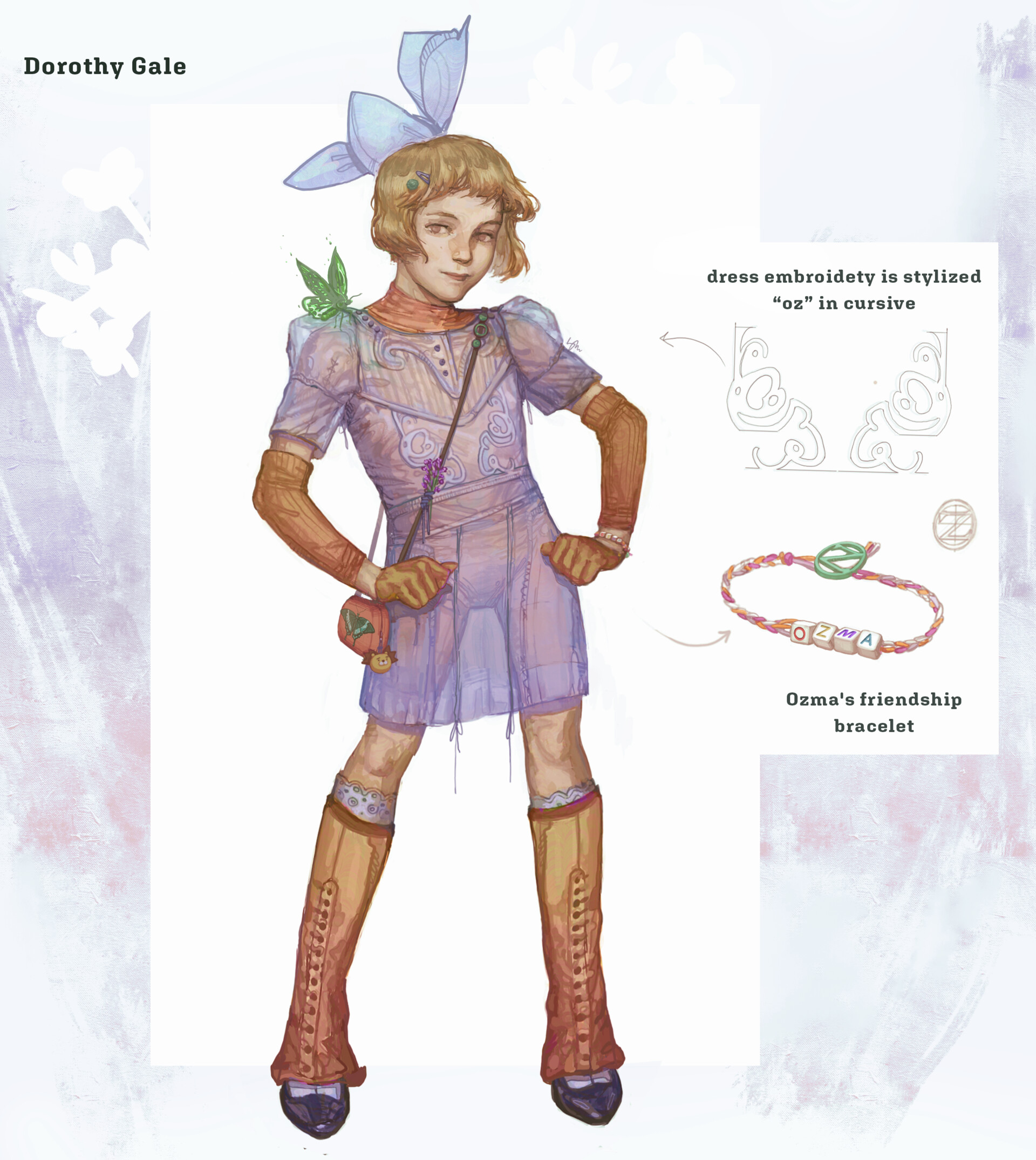The image shows a colorful and detailed artwork of a young girl standing confidently with her arms on her hips. She appears to be around 7 or 8 years old, with short blonde hair adorned with a purple bow tie. She is dressed in a sheer purple fairy-like dress through which an orange shirt and matching pants can be seen, along with buttoned-up orange and red leggings. Her outfit is completed with black dress shoes visible below the leggings. The girl is shown in a three-quarter view, gazing ahead with a slight, curious smile on her face. On her right shoulder, a green butterfly is delicately perched. The name "Dorothy Gale" is displayed in the top left corner of the image, and along the right side, it is noted in cursive that the dress embroidery is stylized as 'Oz.' Below this, there is a reference to "Ozma's Friendship Bracelet." The overall style gives a whimsical, fairy-like feel to the character, reminiscent of a cartoon pixie.